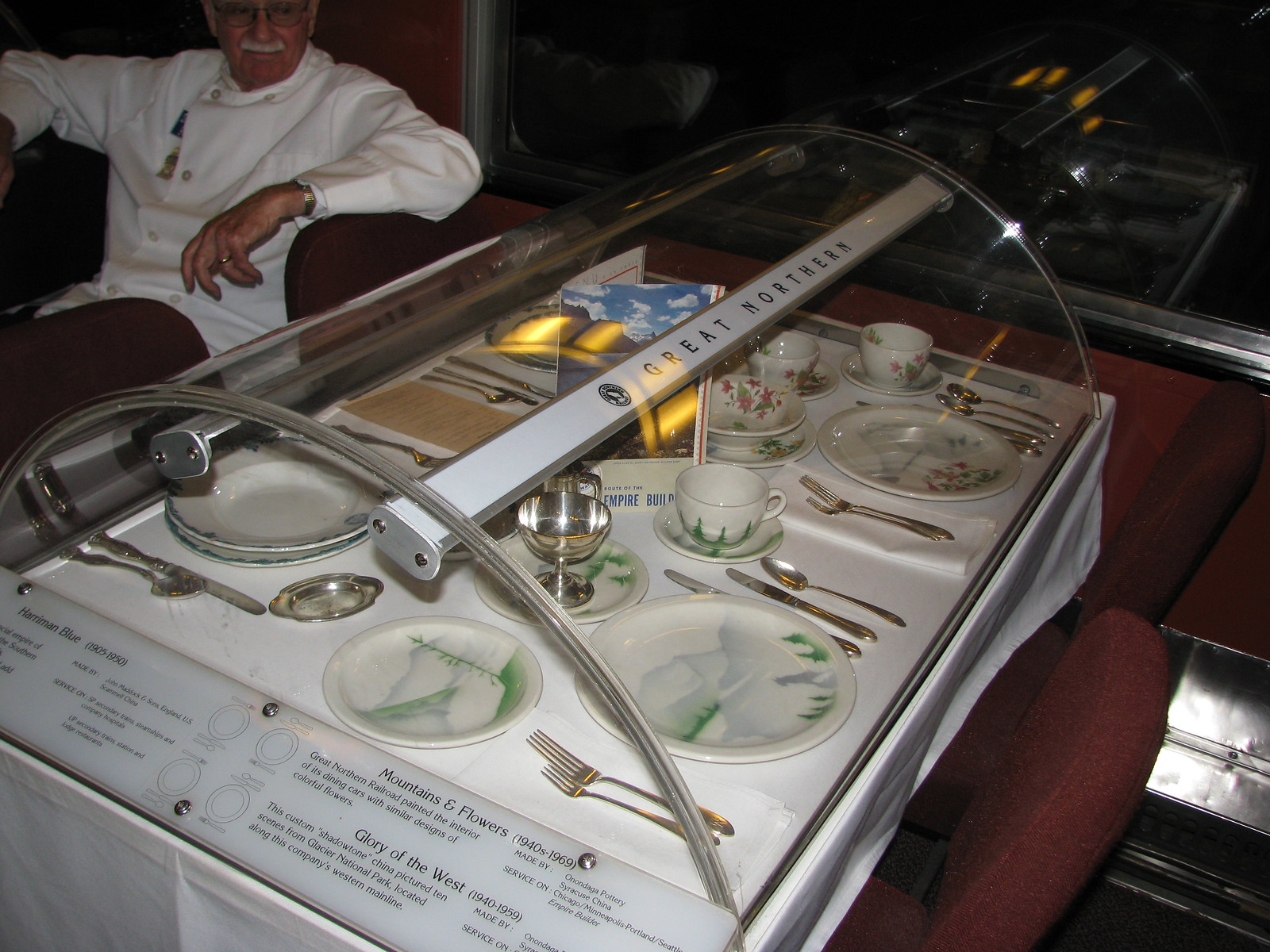The image depicts a meticulously arranged historical display featuring a dining table encased in a rounded glass dome, labeled “Great Northern.” The table is set with plates and silverware, each piece showcasing intricate designs with motifs of mountains, trees, and flowers, reminiscent of the décor used in the Great Northern Railway dining cars. The dome is supported by an internal bar also marked “Great Northern,” with open ends at the sides. 

Accompanying the table setting are silver cups and utensils, enhancing the exhibit’s vintage railway dining experience. Detailed plaques describe the origins and themes of the displayed china, such as the “Mountains and Flowers” set from the 1940s to 1969, and the “Glory of the West” custom shadow tone china, which depicts scenes from Glacier National Park. Another noted design is the “Harriman Blue” china, dated from 1905 to 1950.

The display is set up like a dining scene, complete with a tablecloth and surrounding seats, inviting viewers to imagine the bygone elegance of railway dining. Positioned nearby, a man with a gray mustache and a white sweater is relaxing, adding a human element to the historical tableau. This extensive exhibition highlights the detailed craftsmanship and historical significance of the Great Northern Railway’s dining aesthetics.